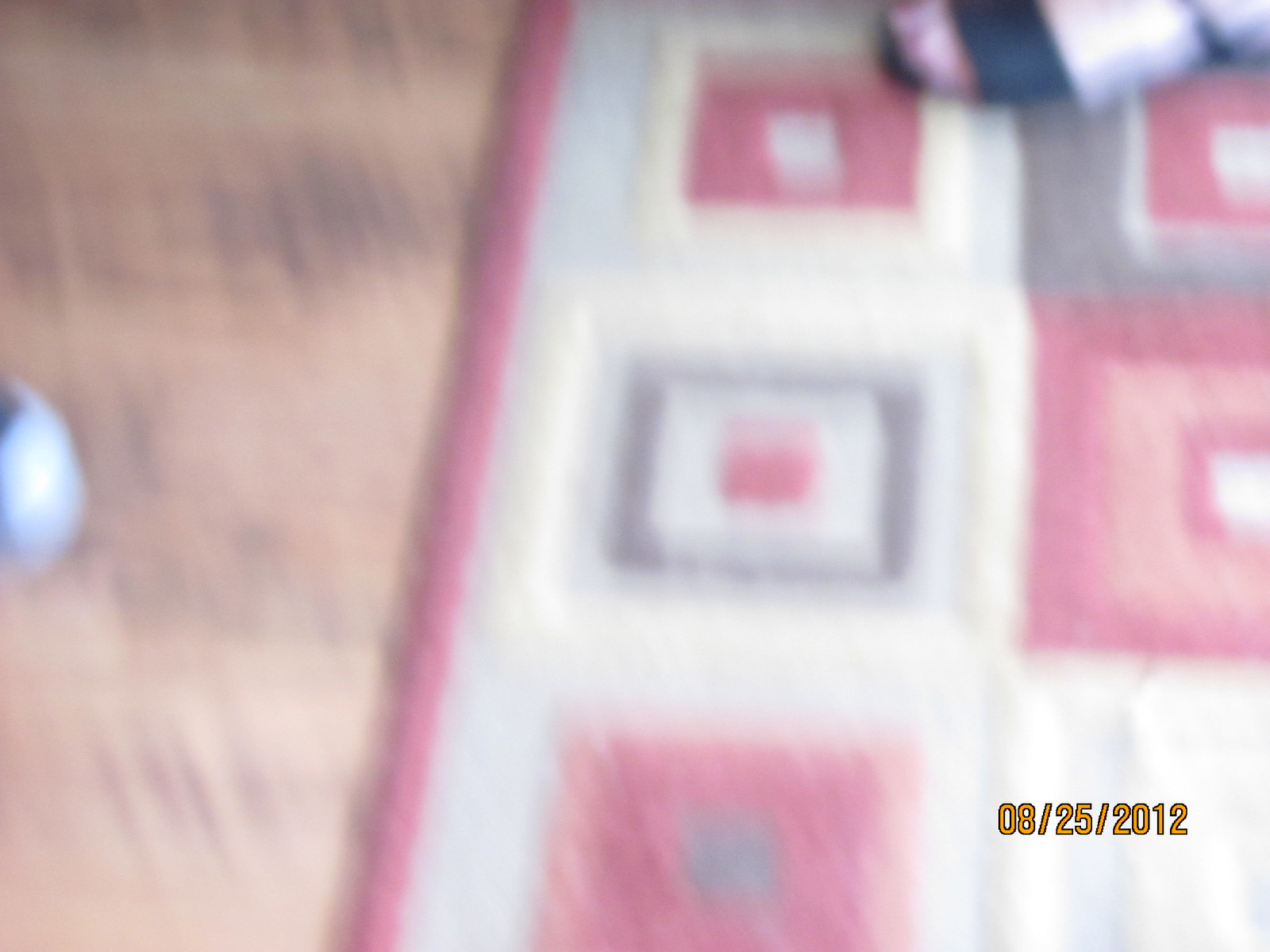In this blurry photograph, a quilt featuring a patchwork of medium blue, dark blue, and red squares, trimmed in red, is spread out on a medium light brown wooden floor. To the right, a partially visible container, likely a blue bowl filled with dog food, is cut off by the frame. The lower right corner of the image reveals a woman's foot adorned with red nail polish. Her foot is strapped in a sandal with a large strap near the toes and a smaller strap around the ankle. A time stamp in gold at the bottom right reads "8/25/2012".